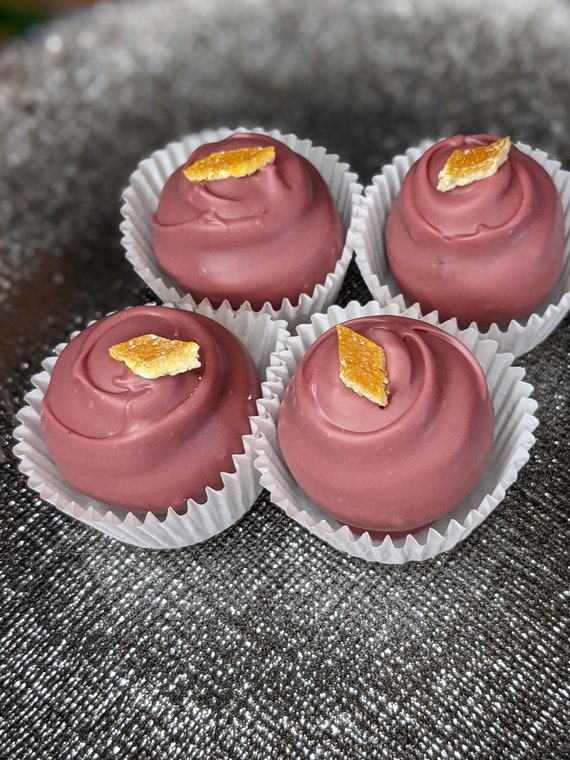The image showcases a close-up view of a stylish food display in portrait mode, featuring four delectable cupcakes prominently placed at the center of a table. The table is adorned with a dark gray fabric tablecloth speckled with silver and white dots. The focus of the image is on the cupcakes, each nestled in double-layered white paper cups. These cupcakes are topped with a smooth swirl of dark pink frosting, leaning towards a light maroon hue. Accentuating the peak of each cupcake is a golden, diamond-shaped pastry or candy. These diamond garnishes have a creamy bottom with a brown top, adding a touch of elegance to the display. The soft focus background further enhances the central appeal, making the cupcakes look irresistibly delicious and drawing viewers' attention directly to them.